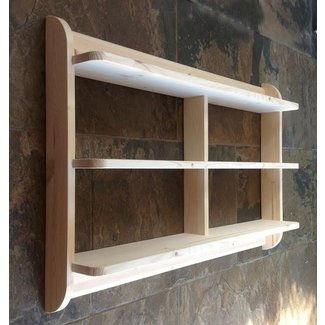This square-format color photograph features a light-colored, three-tiered wooden shelf mounted on a dark gray stone masonry wall. The rustic wall, marred by prominent rust stains, particularly stands out behind the shelf due to its open-backed design. Additional rust marks are visible above and to the left of the shelving unit. The shelves are framed by vertical wooden pieces that elegantly curve at the top and bottom, with horizontal boards securing the top and bottom shelves. The image captures the shelf diagonally from the left, creating a narrowing perspective towards the right. The bottom right corner of the wall is illuminated by sunlight, suggesting an outdoor setting. The wood appears bare and unfinished, adding a handcrafted, personal project feel to the piece.